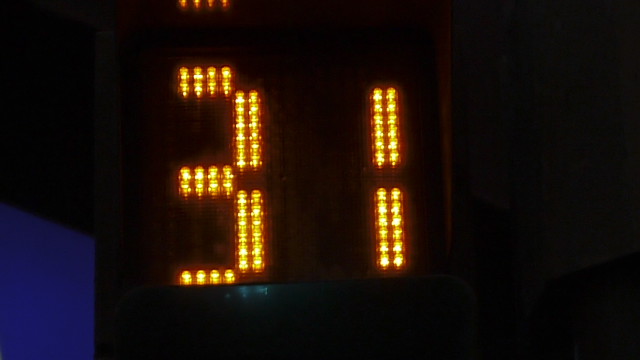This photograph features a black light-up sign prominently displaying the number "31," created using individual LED bulbs arranged in rows of two to form the digit shapes. The LED lights emit a yellow-orange glow, producing a striking contrast against the dark sign. The surrounding background is almost entirely black, with the exception of a noticeable blue square located in the lower-left corner. Reflections add depth to the image: four small orange reflections mirroring the upper stroke of the "3" are visible on the top edge of the sign, and a subtle blue light reflection can be seen beneath the digit "3," likely cast by the wall behind the sign. The overall presentation is highly photorealistic, and the photograph maintains a horizontal rectangular orientation.